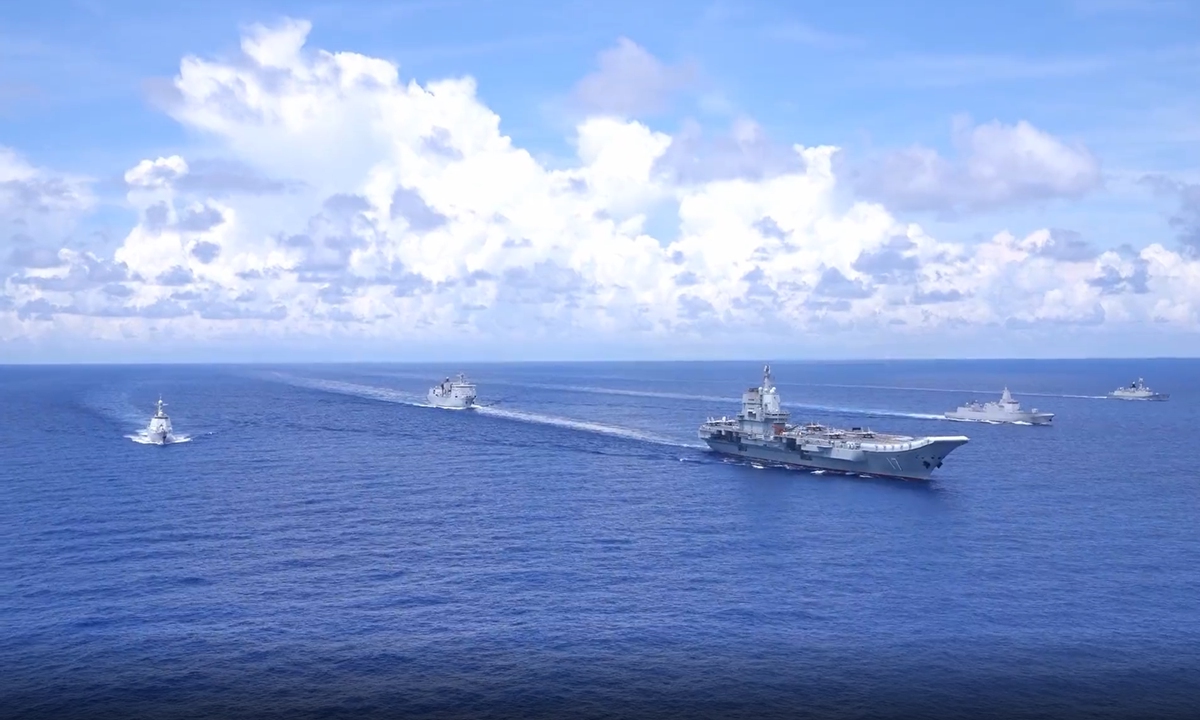This image captures a striking naval fleet traversing the vast and deep periwinkle ocean. Dominating the scene is a massive aircraft carrier, located toward the front of the formation, its immense size emphasizing the smaller stature of the four accompanying ships. The aircraft carrier, with its extensive runway, underscores its military purpose and stature. The formation of five vessels appears to be moving diagonally from the back left to the front right of the image. A brilliant, clear blue sky with a few scattered, large, fluffy white clouds provides a serene contrast to the imposing naval display. The unique interplay of scale between the towering aircraft carrier and its escorting ships highlights the powerful presence of the fleet as it cuts through the wide blue expanse of the ocean.